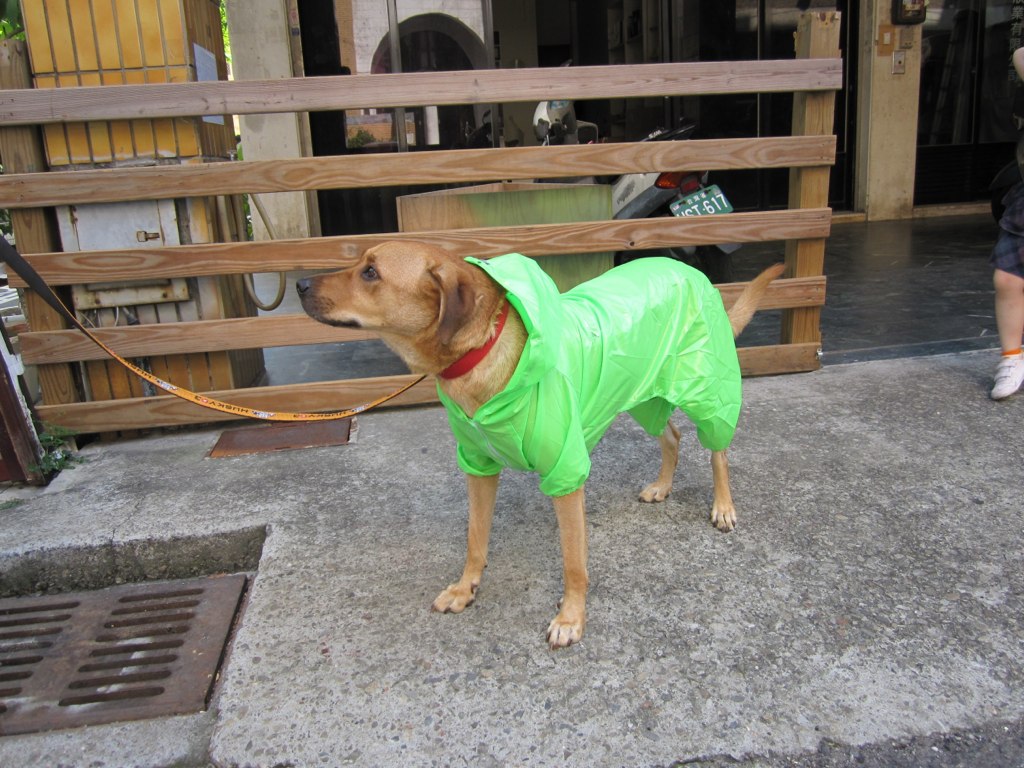In this outdoor photograph, a brown mutt, resembling a beagle, is seen standing on a grey cement pathway adorned with a lime green raincoat made of plastic, reminiscent of a bright green garbage bag. The dog sports a red collar and an orange leash, with its floppy ears draping down and a hood pushed back, revealing a dark nose, black eyes, and a darker brown muzzle. The image captures the dog from its left side, with a profile view of its long tail and a hint of white on its feet.

The background reveals a scene with a brown wooden fence featuring thin, long boards and a wooden post extending to the right. Behind the fence, one can spot a motorcycle with a teal license plate displaying the number 617 in white. To the left of the motorcycle, there appears to be an off-white electrical panel with a lid, and a dark grey rainwater drain is visible at the bottom left. A person’s leg wearing a white shoe, orange sock, and grey shorts appears in the right-hand corner. The surrounding area includes a sidewalk, a potential storefront with a glass window, and a small patio space, adding to the bustling, yet intimate, urban setting.